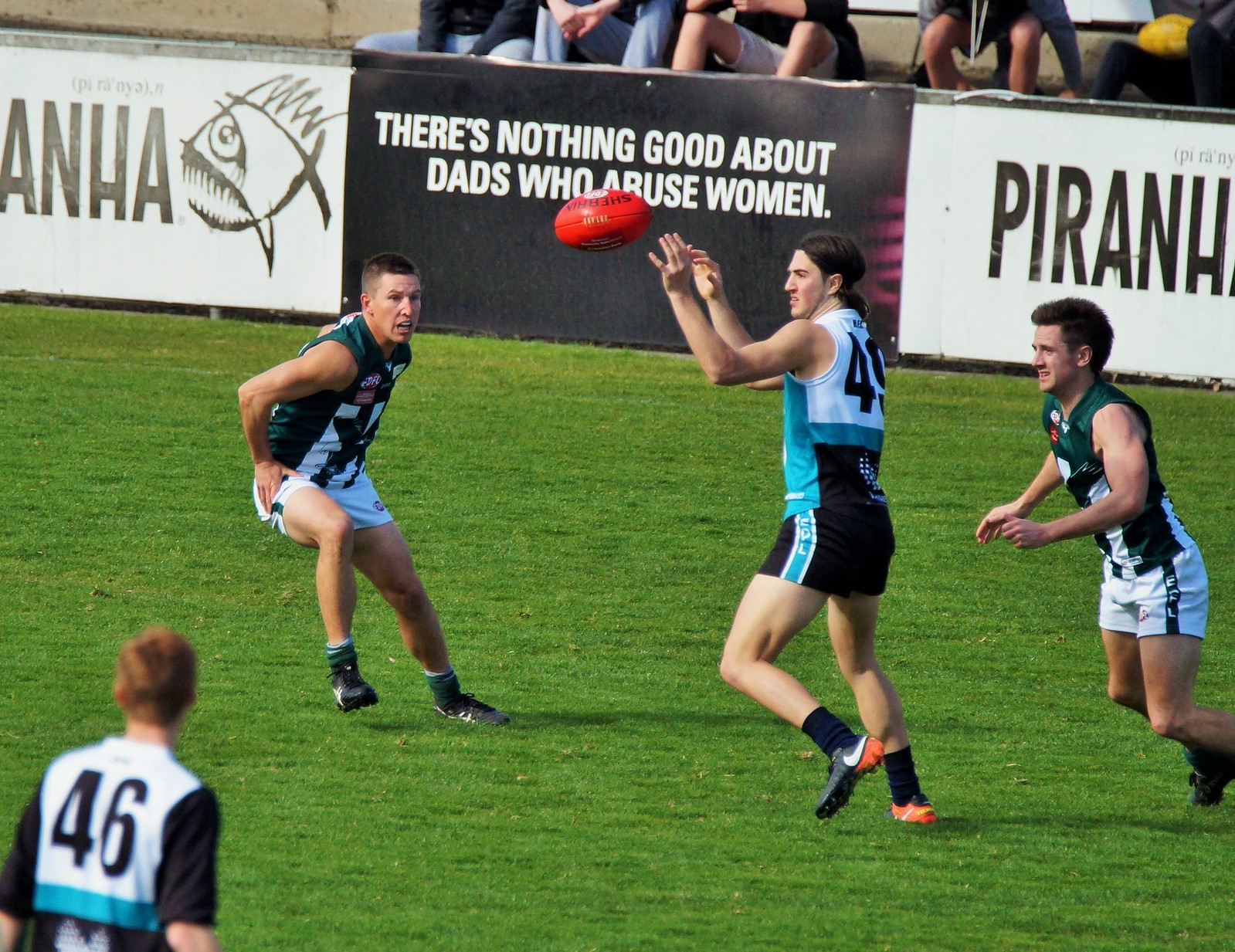In an outdoor photograph taken on a slightly sunny day, four men are playing football on a grassy field. Two of the players are wearing black and white attire, while the other two are in green and white. The focal point of the image is a man with a teal, white, and black jersey, number 49, and black shorts, who is about to catch a red football. This player, who has long brown hair tied in a ponytail, is closely pursued by two players in green and white, seemingly defensive linemen. In the background, a fence adorned with various sponsored ads runs from the top left to the mid-right. The ad on each end of the fence features the word "Piranha" in all caps, accompanied by a sketch of a fish with a large eye. Centrally positioned on the fence is a striking sign with a black background and bold white font that states, "There's nothing good about dads who abuse women." The image captures a dynamic and tense moment in the game, with the vivid advertisements in the background adding to the scene's intensity.